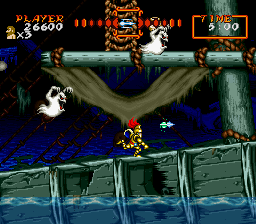In this dynamic video game scene, a player in gleaming gold armor races across the deck of a large, gray ship that towers over a body of water. The ship is equipped with colossal masts, including a prominent crossbeam. The player appears to have scored 26,600 points and has three lives remaining, indicated by a '5' and '9' at the top of the screen. The scene is fraught with danger as two ghostly apparitions pursue the armored character—one from beneath the deck and another atop the highest mast. In the distance, a small cloud hovers above the water, adding to the surreal atmosphere.